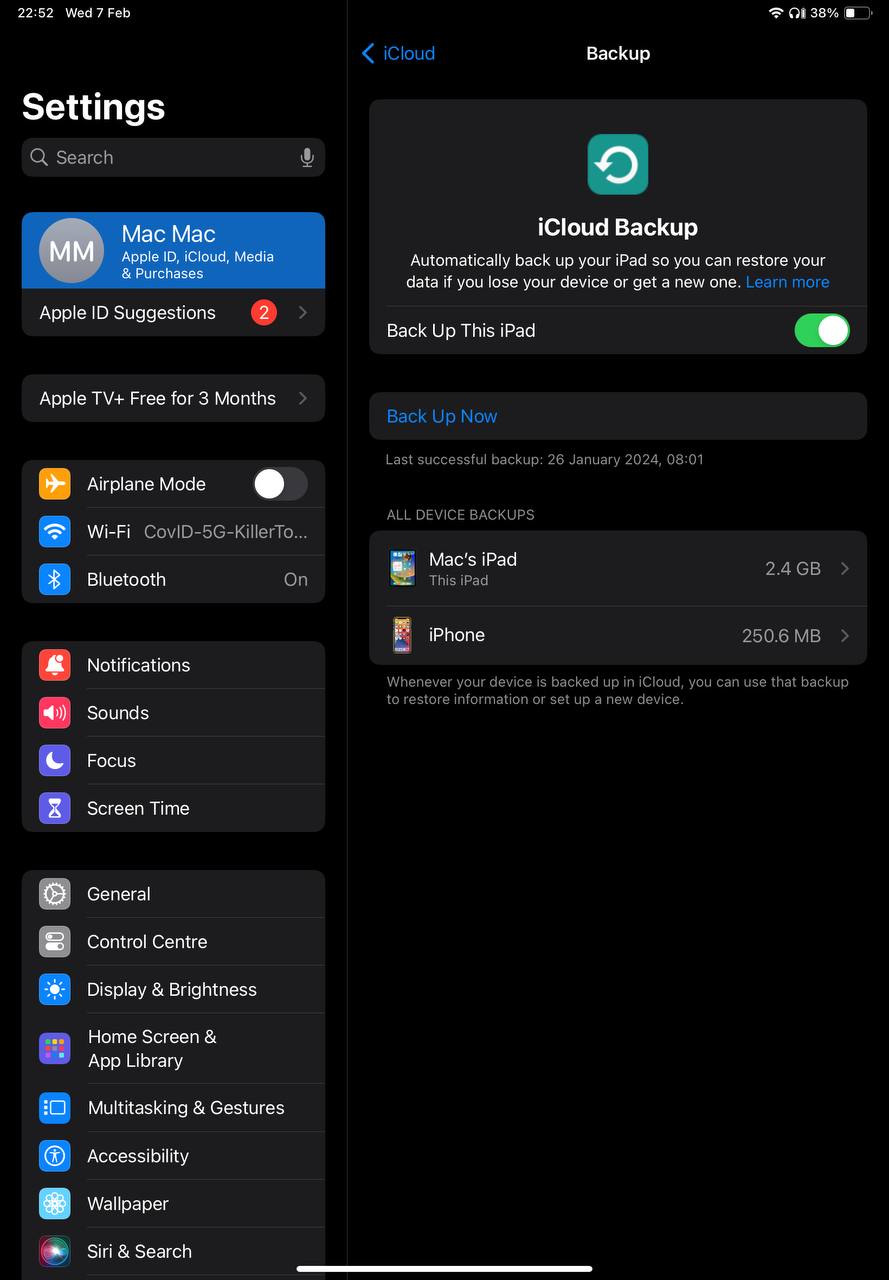The image depicts a detailed view of a settings web page with a dark theme, featuring a mix of colorful icons and white text. At the top, a banner displays the timestamp "22:52, Wednesday, 7 February." To the right of this banner, there are icons for headphones, Wi-Fi, and a battery icon indicating a 38% charge.

Below the banner, a blue left-facing arrow labeled "iCloud" is situated next to the white text "Backup." Directly beneath this is a black box featuring a refresh icon and white text that reads, "iCloud Backup: Automatically backs up your iPad so you can restore data if you lose your device or get a new one. Learn more."

Continuing down the page, a toggle switch for "Back up this iPad" is turned on, with a "Back up now" button positioned below it. The last successful backup is noted as "26 January, 2024, 8:01."

The list of device backups includes "Mac's iPad" and an "iPhone." To the left of this section is a navigation path labeled "Settings," followed by a search box equipped with a microphone icon.

Next on the page are various account and service details, starting with "MM, Mac, Apple ID, iCloud, Media and Purchases." Below this, "Apple ID Suggestions" shows two suggestions with a right-facing arrow, followed by "Apple TV Plus, free for three months."

Further down, the page features an airplane mode icon with the mode turned off, and details about the current Wi-Fi network "COVID-5, 5G killer 2," with Bluetooth listed as "on."

The settings page continues with icons for Notifications, Sound, Focus, Screen Time, General, Control Center, Display and Brightness, Home Screen and App Library, Multitasking and Gestures, Accessibility, Wallpaper, and Siri and Search.